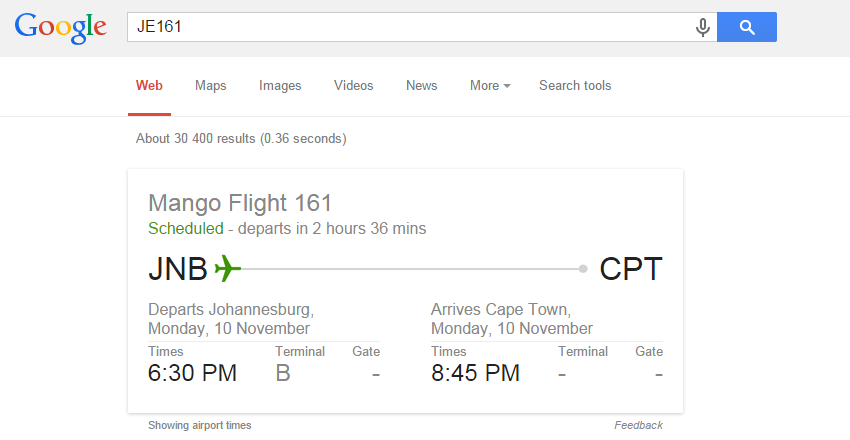The image captures a screen from a desktop computer displaying a Google search results page. The interface features a predominantly white background. Positioned in the upper-left corner is Google’s iconic, colorful logo. Adjacent to the logo is the search bar, containing the input "JE161." On the right side of the search bar is a blue search button icon.

Below the search bar, the navigation menu for different types of search results is visible. The "Web" option is highlighted in red and underlined, indicating it is the selected category. Other options listed from left to right include "Maps," "Images," "Videos," "News," "More," and "Search tools."

Further down, the screen notes that there are approximately 30,400 results found in about 0.36 seconds. The screen shows a detailed search result, specifically for "mango flight 161." This search result appears to be the primary focus of the user's query.